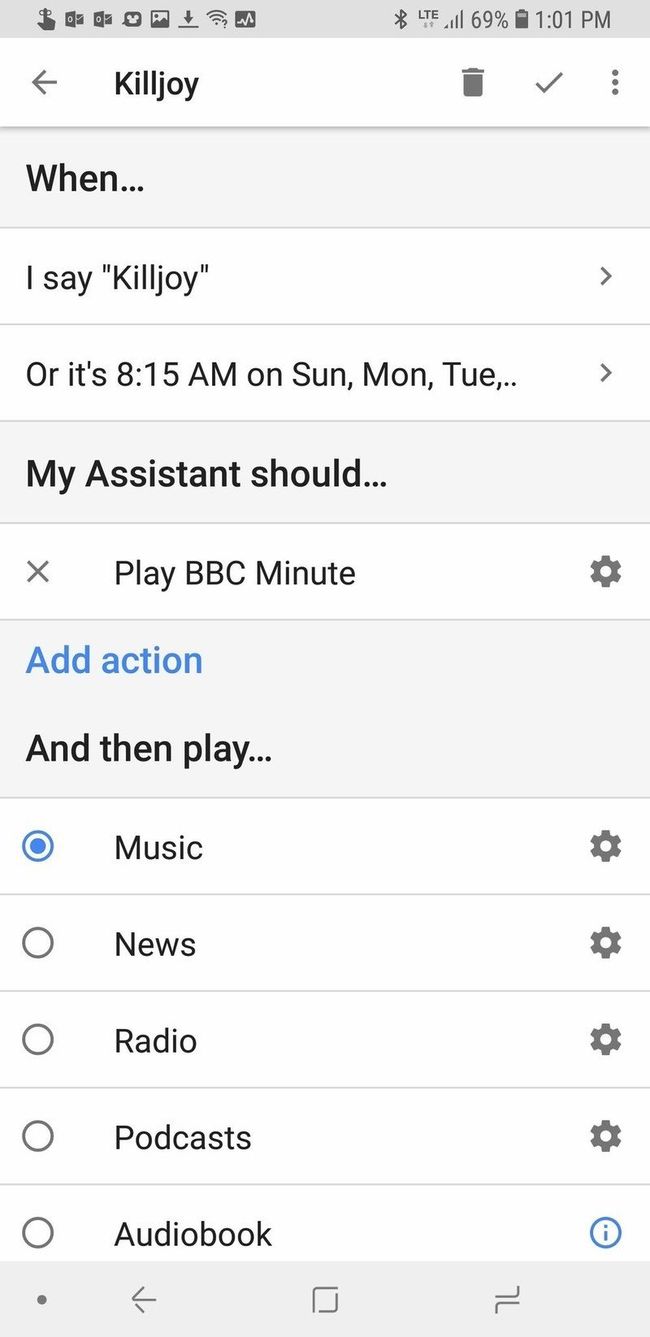This rectangular portrait image appears to be a screenshot taken from a cell phone. The interface resembles a settings page, possibly from a mobile application or a task automation tool. The layout features roughly ten rows, with alternating gray and white backgrounds. Except for a few blue elements, the image primarily uses black and white hues. 

At the very top is a light gray header, which is not very tall. This section contains eight icons in total, distributed on both the left and right sides. The left side features icons such as a hand pointing upwards with a circular outline at the fingertip, a download icon depicted as a downward arrow over a line, and a Wi-Fi signal icon that looks like three curved lines forming a pie slice. On the right, there are more icons like a signal strength indicator with four ascending bars, a numerical battery percentage reading at 69%, and a vertical battery icon showing three-quarters full. Additionally, the time reads 1:01 PM on the far right.

Below the header is a white bar containing a leftward-facing arrow followed by the text "Killjoy" on the left side. On the right side of this bar, there are three icons: a garbage can, a checkmark, and three vertical dots.

The next section features a light gray background with the text "When..." in darker gray on the left. Below this, two white fields are separated by thin gray lines. The first field reads: "I say 'Killjoy'" and the second specifies a time: "8:15 a.m. on Sun, Mon, Tue...". Both fields have rightward-facing arrowheads on the far right.

Following this is another gray section labeled "My assistant should...", identical in format to the previous gray row. Beneath this, there’s a white field with a grey X on the left, text that reads "Play BBC Minute," and a gear icon for settings on the far right.

The next gray section is twice as tall as the others. It contains medium blue text that says "Add action" in the upper left corner, followed by black text "and then play...". Five white fields are listed below, each with a corresponding radio button on the left. The options are "Music", "News", "Radio", "Podcasts", and "Audiobook". The first radio button is filled in blue with a blue outline, while the others are gray. The first four rows have the settings gear icon on the right, and the audiobook row has a blue information icon.

At the bottom of the image is another light gray background containing four dark gray icons: a small dot, a leftward-facing arrow, an incomplete square, and two parallel lines resembling hockey sticks where one curves upwards and the other downwards.